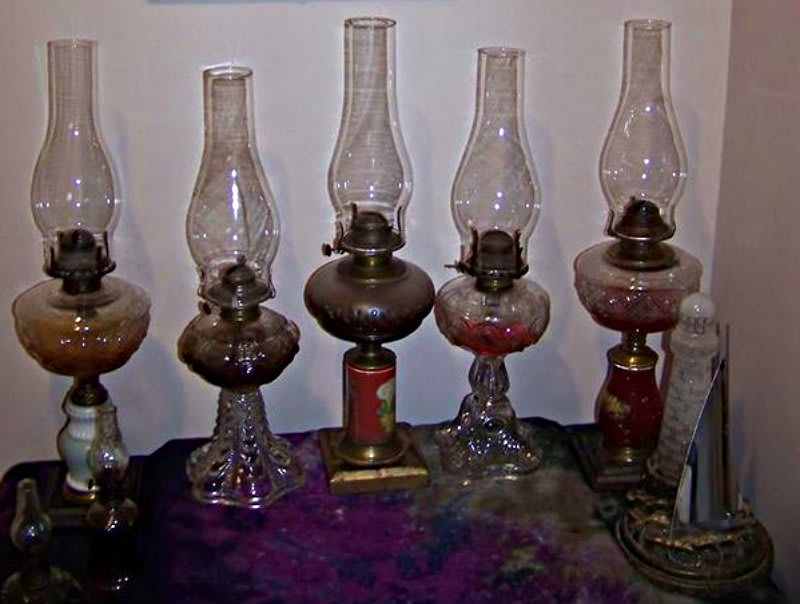In this image, we see a collection of five ornately designed oil lamps, arranged in a slightly landscape perspective on a purple tablecloth with a white wall as the backdrop. The lamps vary in style and material, showcasing a vintage charm and appearing to be heavily used. The bases differ among the lamps: the one on the left has a white ceramic base, while the middle and rightmost lamps feature red bases. In contrast, the second and fourth lamps from the right boast glass bases shaped in a seashell-like design. All the lamps have a wide glass canister in the middle, except for the central lamp, which has a metal canister likely meant to hold torch fuel. Each lamp is topped with a tall, thin glass flume where the flame is captured. The glass components of the lamps have a bulbous shape, expanding at the bottom and tapering off at the top, resembling antique glassware used over fifty years ago. They are characterized by their worn appearance, indicative of extensive use, adding to their historical aesthetic.